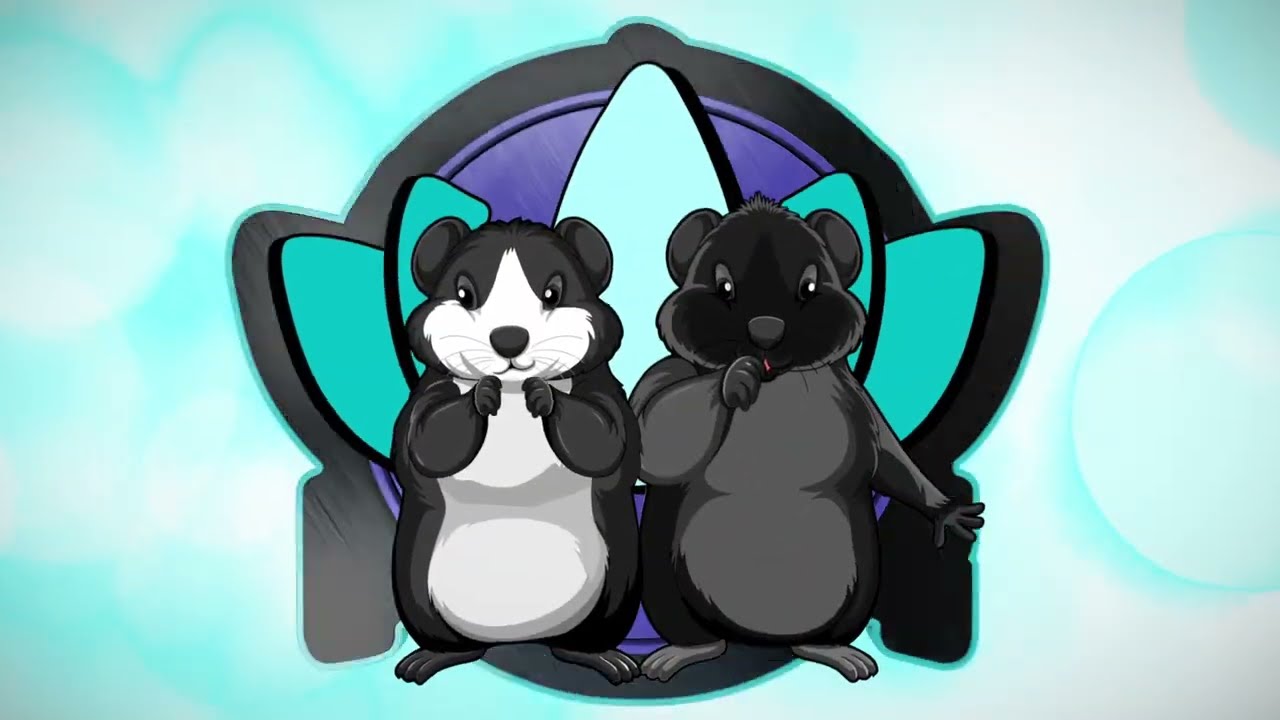In the digital artwork, two charming gerbil-like creatures take center stage. The one on the left resembles a panda with a white belly, white face, and black exterior, including black arms and ears. The creature on the right has a darker appearance, sporting a black face and a grayish-black body. Both are stylized with digital art, adorned with black eyes and detailed three-toed feet. They are positioned against a backdrop featuring a vibrant emblemific lotus flower, colored in various shades of turquoise and light green. This emblem sits within a purple circle outlined in black. The larger background shifts from a gradient of blues to light turquoise, reminiscent of a sky imbued with bubbles. Both creatures appear to be merrily engaging with the scene, with the right creature playfully placing its left arm against the flower, adding a lively and distinctive touch to the image.